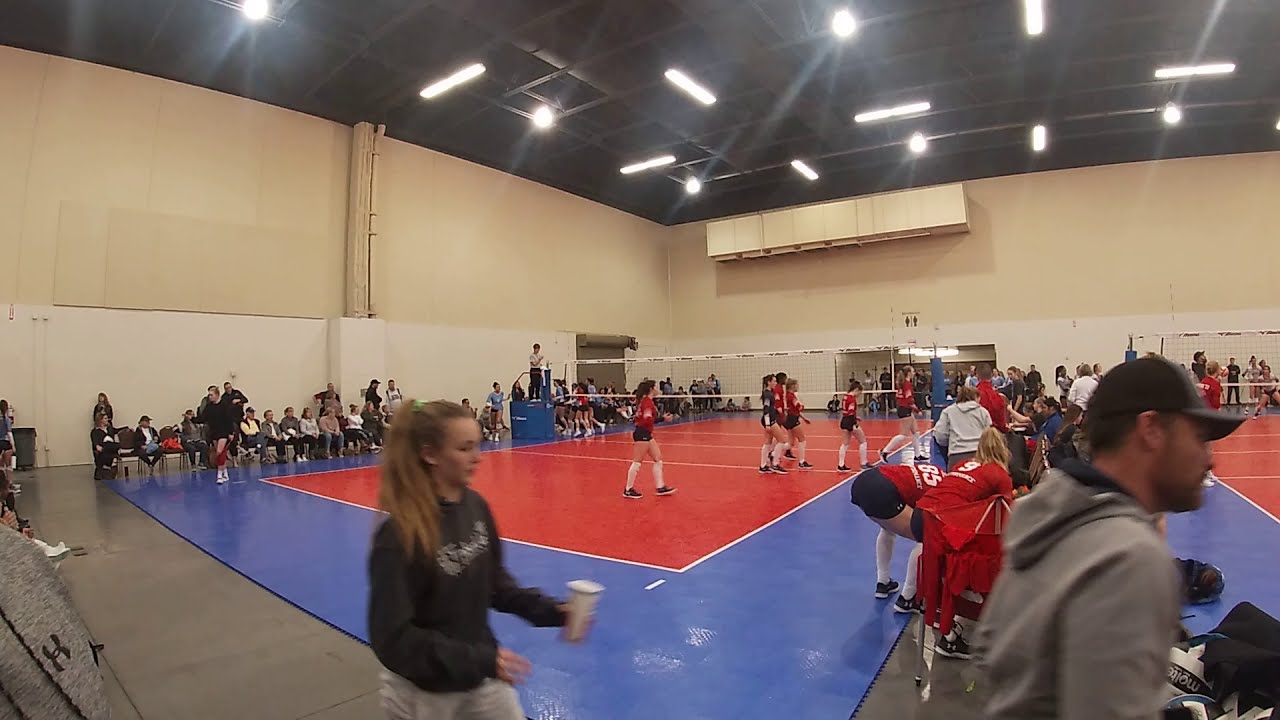The image captures a bustling indoor volleyball game set in a spacious, well-lit gymnasium with a ceiling structured in black steel and adorned with both circular and rectangular white fluorescent lights. The primary feature of the scene is a prominently visible volleyball court with blue edges and a red center, crisply marked with white lines that delineate various areas. A white net with black netting, held up by blue pillars, stretches across the center of the court.

In the foreground, a girl with a ponytail, dressed in a black sweater, is seen holding a cup in her left hand as she walks to the right. Nearby, a man wearing a baseball cap and a grey jacket stands at the right corner of the image.

The far wall of the gymnasium displays a two-tone color scheme with tan on top and white on the bottom. The floor beneath them is solid, polished dark grey concrete. The gymnasium is bustling with activity, featuring multiple people including teams and spectators.

A team in red and black uniforms, black tennis shoes, and tall white socks is actively engaged on the court, while parents and other spectators line the walls and sides, observing the game. The spectators form a line along the back left end, extending towards the center of the main volleyball court and another line behind each visible court on the right. The dynamic and vibrant atmosphere encapsulates a typical, lively volleyball game setting.